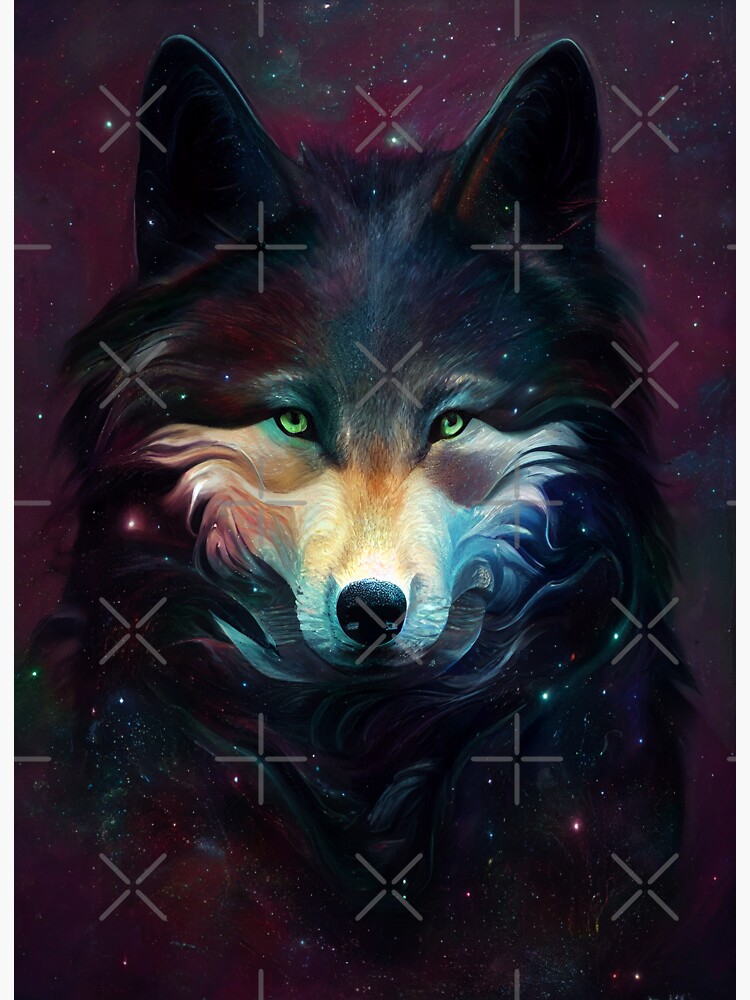The poster features a computer-generated drawing of a solitary black wolf with tall, straight ears and a small black nose. The wolf's muzzle and cheeks are white, as is the area between its nose and eyes, while its nostrils have purplish and orange hues. The wolf's piercing green eyes stare directly at the viewer. The poster's background consists of multiple shades of purple, resembling a starry night sky, with white, shining lights and embedded symbols including stick X figures and cross figures arranged in alternating rows.